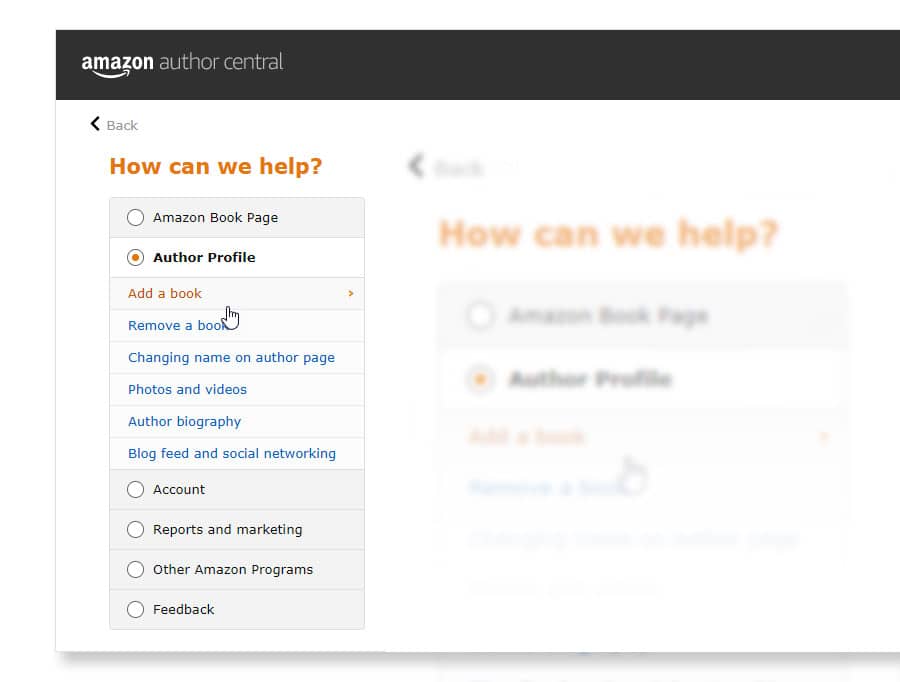The image depicts a webpage from the Amazon website, specifically the Author Central section. At the top of the page, there is a black navigation bar with "Amazon" displayed in white font accompanied by the trademark arrow logo beneath it. To the right, "Author Central" is prominently featured. Below this, a white box dominates the screen.

In the upper left corner of this box, a left-facing black arrow accompanied by the word "back" is visible. Beneath this, the text "How can we help?" is displayed in mustard-colored font.

A vertical gray sidebar lists several categories, each accompanied by a selection circle. The categories are:

1. **Amazon Book Page**
2. **Author Profile** (selected, with a mustard dot in the circle)

Subcategories related to the "Author Profile" are listed below, all in blue font except for the selected subcategory, which is in mustard font:
- Add a Book (selected)
- Remove a Book
- Changing Name on Author Page
- Photos and Videos
- Author Biography
- Blog Feed
- Social Networking

Additional categories (unselected) include:
- **Account**
- **Reports and Marketing**
- **Other Amazon Programs**
- **Feedback**

To the right of the sidebar, a ghosted overlay enhances the visual, showing partially transparent elements for the back button, "How can we help?" text, and the first two categories: Amazon Book Pages and Author Profile.